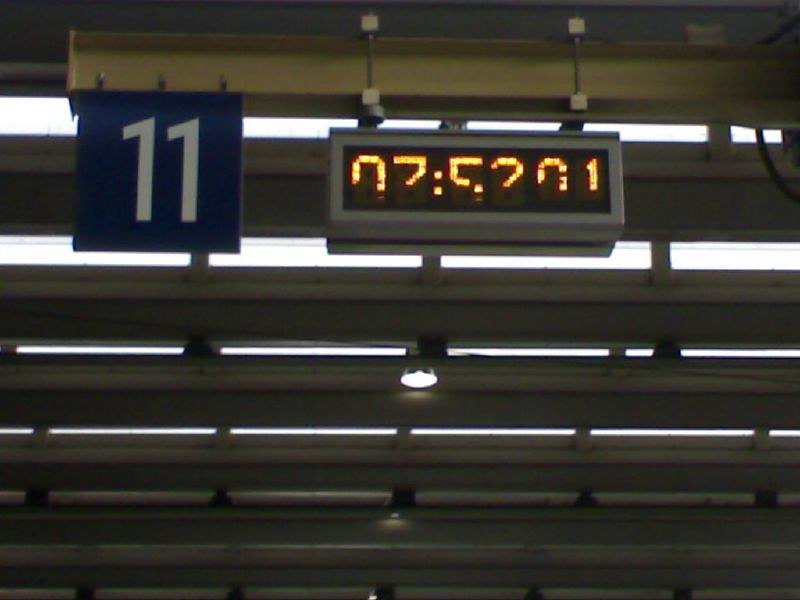The image depicts a ceiling, possibly in a commercial setting like a store, featuring built-in white strip lights that run along its length. A central beige post extends from the ceiling, supporting a large blue box with a prominent white number "11" displayed on it. Additionally, a rectangular device resembling a digital clock hangs from the top of the same post. This device has an off-white trim and a dark center, displaying partially illuminated numbers "07:5201" where the bottom half of each character is not lit. The ceiling is further adorned with evenly spaced round lights, all of which are illuminated, providing ample lighting throughout the area.